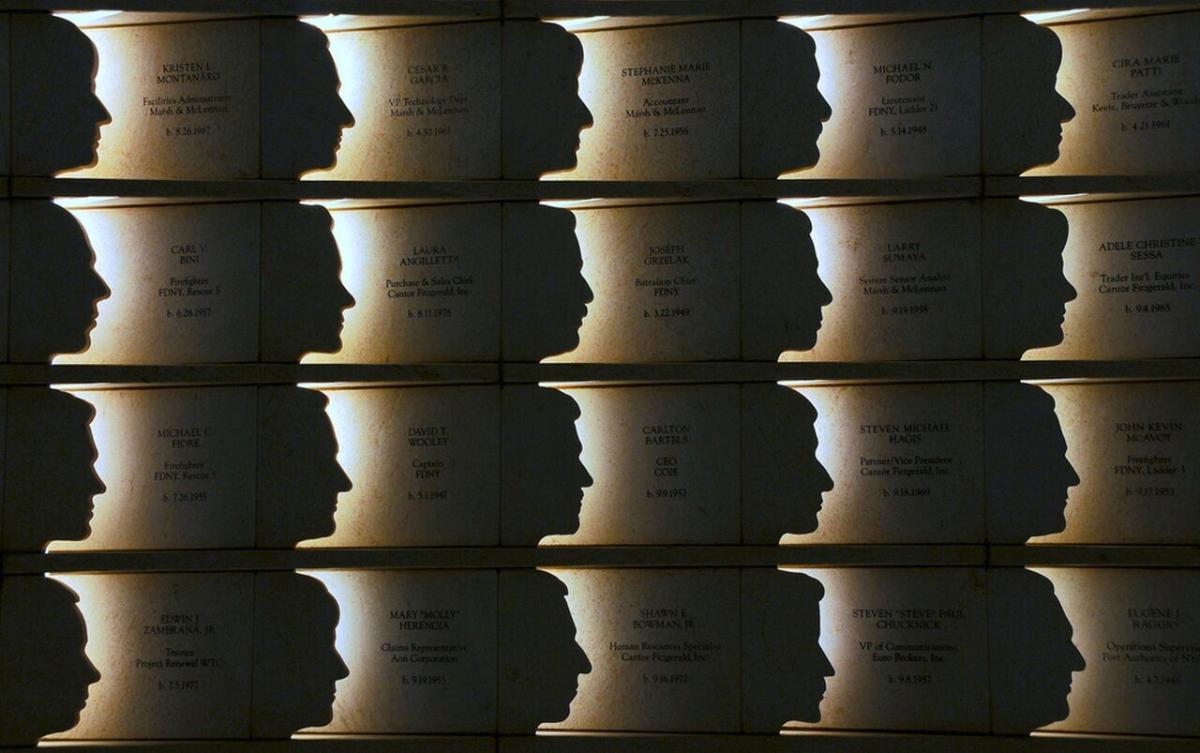The image is a poignant collection of 20 small square silhouettes arranged in a 4x5 grid, each depicting a side profile of a person looking to the right. Illuminated by a soft light from behind, these silhouettes cast a glow on brief, typed information next to them, including names and possibly titles, though the text is too small to fully decipher. The individuals vary between men and women, with names like Kristin Montanar, Caesar, Stephanie, Michael Odor, Carl, Laura, Joseph, Larry, Adele, Michael, David, Carlton, Stephen, Edwin, Mary, Shawnee, and Sean being partially readable. This collection resembles a tribute wall, potentially honoring fallen New York Fire Department employees, characterized by the somber and respectful presentation of their profiles and names, yet devoid of clear birth or death dates.